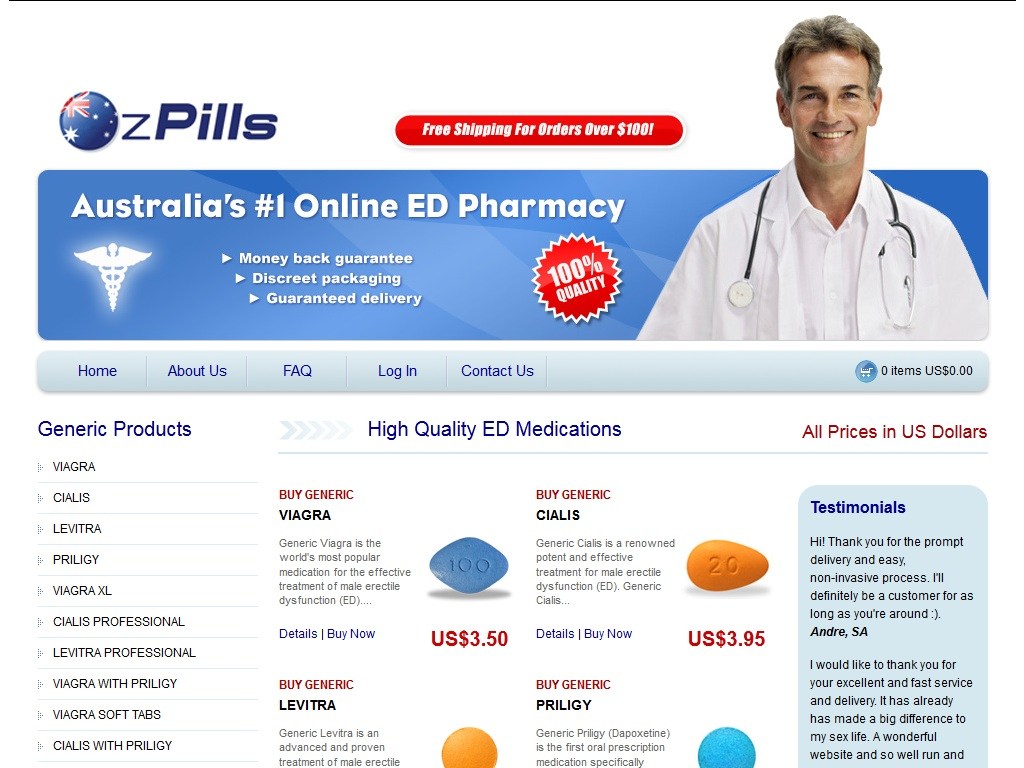The website for Z Pills, a prominent online pharmacy specializing in erectile dysfunction (ED) medications, features a visually appealing and informative homepage. At the top, the company's name, "Z Pills," is displayed prominently beside their logo: a navy blue round ball adorned with various stars, resembling elements of the UK flag.

A striking orange box highlights an attractive offer: "Free Shipping for Orders Over $100." Below this, an image of a smiling pharmacist, who may also be a doctor, is shown. He has graying hair, wears a white lab coat, and has a stethoscope draped over his shoulders, adding a professional touch.

The website proudly touts itself as "Australia's Number One Online ED Pharmacy," emphasizing key benefits such as a money-back guarantee, discrete packaging, guaranteed delivery, and 100% quality assurance. This information is underscored by a circular orange badge with white lining, featuring the classic medical symbol with a serpent and wings.

Navigation through the site is user-friendly with a light gray menu bar containing links to "Home," "About Us," "FAQ," "Login," and "Contact Us." The shopping cart icon, indicating zero items, is located near the top right corner.

The homepage offers a catalog of high-quality generic ED medications, with prices displayed in US dollars. Some featured products include generic Viagra, Cialis, Levitra, and Priligy. Testimonials, located in a blue box on the right side of the page, provide customer reviews and experiences, adding credibility and trustworthiness to the site.